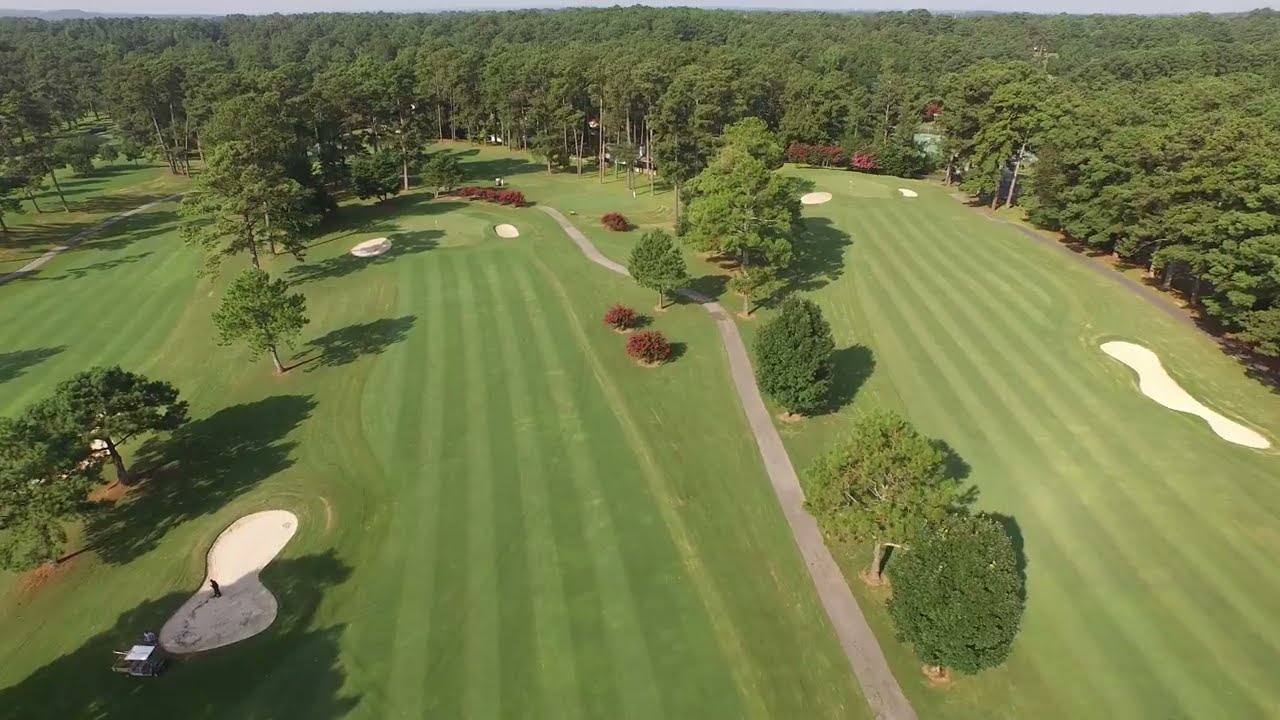This image is an aerial photograph of a lush, green golf course taken from a drone, giving a high-angle view of the landscape. Dominating the center of the image is a roadway that leads up from the bottom, flanked by a meticulously maintained putting green. The fairways are lined with tall trees, including varieties like eucalyptus and pine, creating a verdant and picturesque scene. To the far right, a white clubhouse with a striking red tile roof is clearly visible, along with several nearby buildings. Scattered across the course are various sand traps and bunkers, their brownish hues contrasting with the immaculate greenery. In the middle of the image, there's a distinctive patch of reddish vegetation, likely flowers or ornamental plants, adding a splash of color. The image also captures two golfers mid-game near a cart, with one by the green surrounded by similar reddish plants. The overall scene is sunlit and bright, indicating it was taken outdoors in the middle of the day.